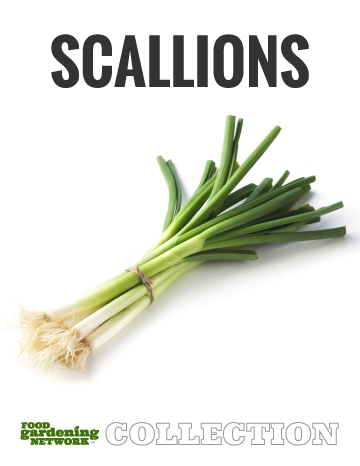This image depicts a neatly bundled bunch of scallions, prominently displayed against a pure white background. The scallions, held together by a tan rubber band, transition in color from their white roots at the bottom to light green in the middle and dark green at the tops, which are uniformly cut. The bundle contains roughly 4 to 8 scallions, all in pristine condition. At the top of the image, bold black uppercase letters spell out "SCALLIONS." Below the scallions, the text "Food Gardening Network" is featured in green, accompanied by the word "Collection" in white letters with a black outline. The overall presentation highlights the fresh and vibrant appearance of the scallions while associating them with the Food Gardening Network.